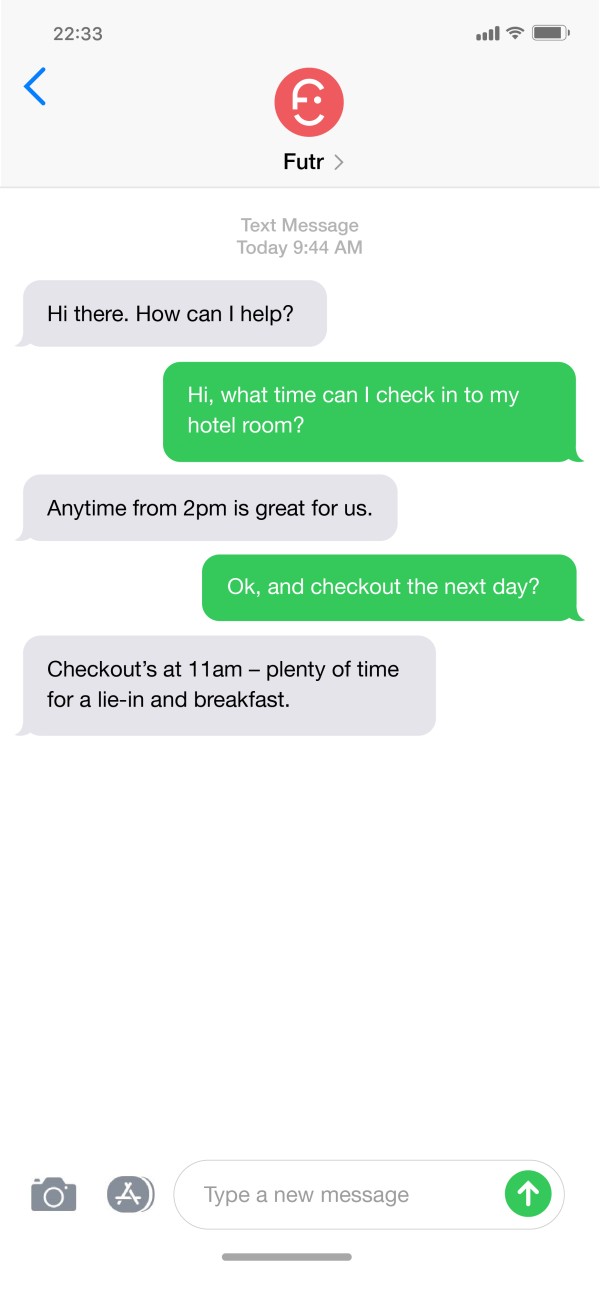This image is a screen capture of a text conversation between two individuals on a smartphone. At the top of the screen, the contact name "F-U-T-R" is displayed, though the origin of this name is unclear. The status bar indicates it is 9:44 AM, and icons show the battery life, Wi-Fi connectivity, and cellphone signal strength.

Below the contact name, it states "Text Message Today 9:44 AM." The conversation reads as follows:
1. "Hi there, how can I help?" (sent by F-U-T-R)
2. "Hi, what time can I check in to my hotel room?" 
3. "Any time from 2 PM is great for us."
4. "Okay, and check out the next day?"
5. "Check out at 11 AM. Plenty of time for a lie-in and breakfast."

Below the conversation, there is a text input field labeled "Type a new message" with a send button located to the right. To the left of the input field, there are two icons: an 'A' symbol, likely for text formatting options, and a picture symbol for uploading or sharing images. At the very top left of the screen, beneath the current time, there is a blue arrow pointing left, presumably for navigating back to a previous screen. Above the contact name, there is a red circle icon with a face symbol, indicating the user’s avatar or profile picture.

Finally, a subtle gray line at the bottom of the screen suggests a handle for scrolling or moving the page within the app.